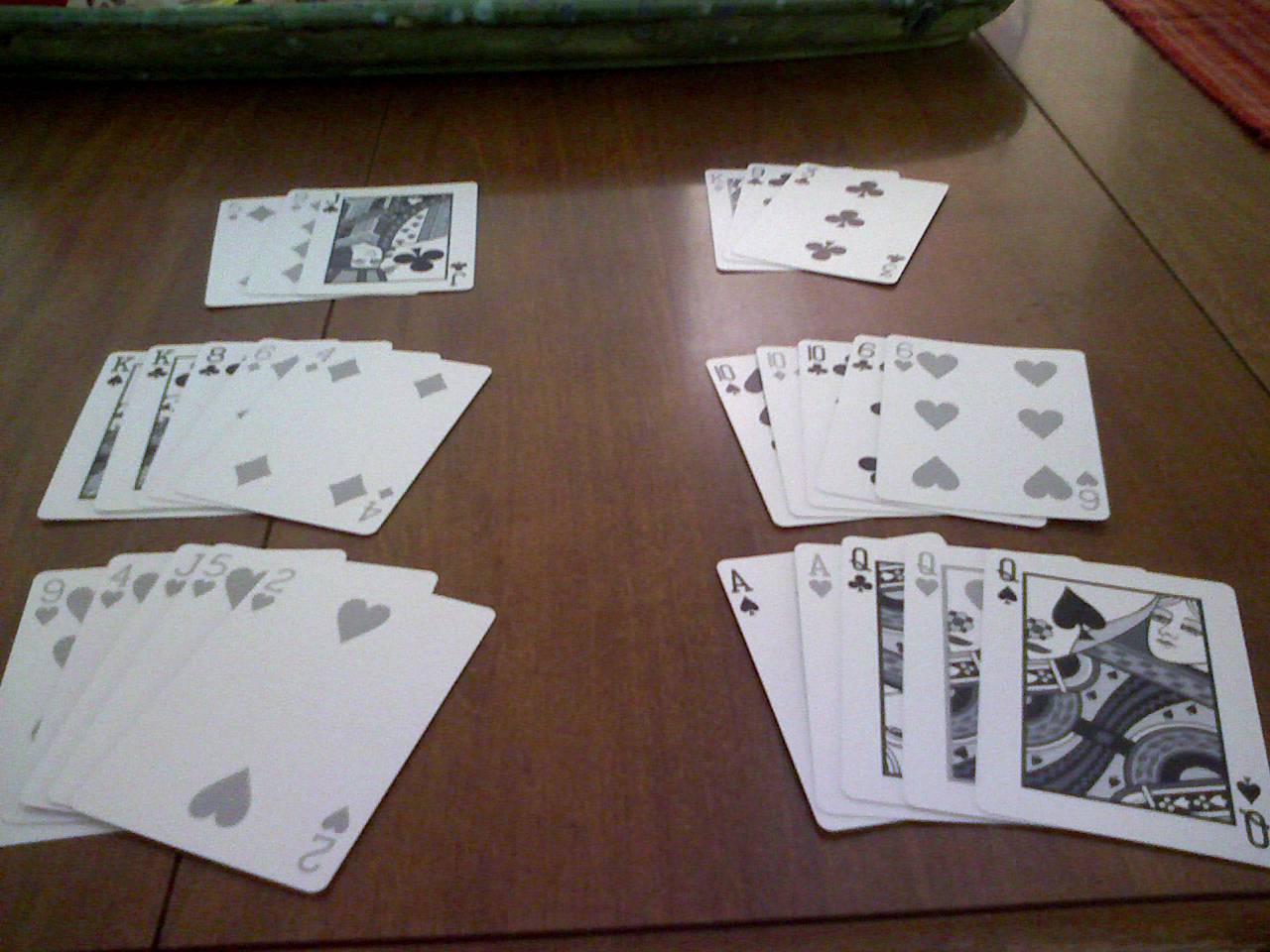The image features a dark brown wooden table neatly displaying several playing cards arranged in two columns. Each column is organized into three distinct sections with a specific pattern: the top section has three overlapping cards, followed by a mid-section of five overlapping cards, and finally, another set of five overlapping cards at the bottom, much like hands of poker.

In the top left section, the cards shown are the Five of Diamonds, Nine of Diamonds, and Jack of Clubs. In the top right section, the three cards are the King of Hearts, Nine of Clubs, and Three of Clubs. 

The middle left section reveals a mixed hand consisting of the King of Spades, King of Clubs, Eight of Clubs, Six of Diamonds, and Four of Diamonds. The middle right section displays a full house made up of the Ten of Spades, Ten of Diamonds, Ten of Clubs, Six of Clubs, and Six of Hearts. 

Moving to the bottom sections, the left side showcases a flush in hearts with the following cards: Nine of Hearts, Four of Hearts, Jack of Hearts, Five of Hearts, and Two of Hearts. The bottom right section exhibits another full house, specifically two Aces and three Queens: Ace of Spades, Ace of Hearts, Queen of Clubs, Queen of Hearts, and Queen of Spades. 

The careful arrangement and the specific hands displayed suggest a poker-themed setup, providing a visually intriguing glimpse into possible game scenarios.